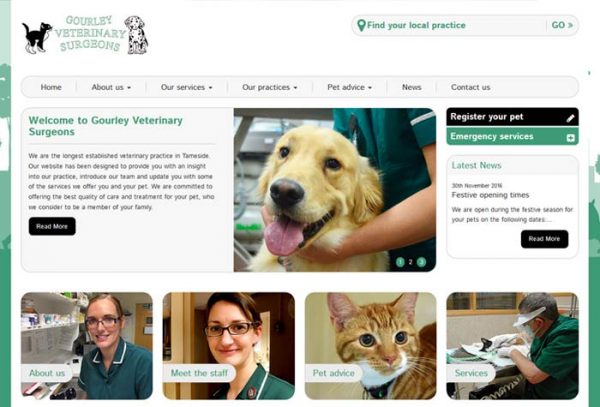The image is a screenshot from a desktop or laptop PC, featuring a widescreen aspect ratio typical of computer monitors. It displays a webpage belonging to Gorley Veterinary Surgeons. The site has a light background accented by a white and green color scheme, with green borders on the left and right sides of the page. Titles of articles and some other text are highlighted in a light green hue. All depicted doctors are dressed in green shirts.

The header of the webpage prominently features the text “Gorley Veterinary Surgeons” in green, accompanied by a small drawing of a cat on the left and a Dalmatian puppy on the right. Adjacent to these drawings is a search bar labeled "find your local practice" in green text, which is paired with a green "Go" button. 

Below the header, there are navigation tabs that read: Home, About Us, Our Services, Our Practices, Pet Advice, News, and Contact Us. Following the navigation tabs, a welcome message declares “Welcome to Gorley Veterinary Services,” accompanied by a paragraph of small black text that is not readable in the screenshot. 

Next to the welcome message is a picture of a cute golden retriever, gazing directly at the camera with its pink tongue playfully sticking out. Beneath this section, there are four images: the first two depict women in green shirts and glasses, smiling at the camera. The third image shows an orange tabby cat. The fourth image features a man, also in a green shirt and wearing a face mask, performing a procedure on a cat.